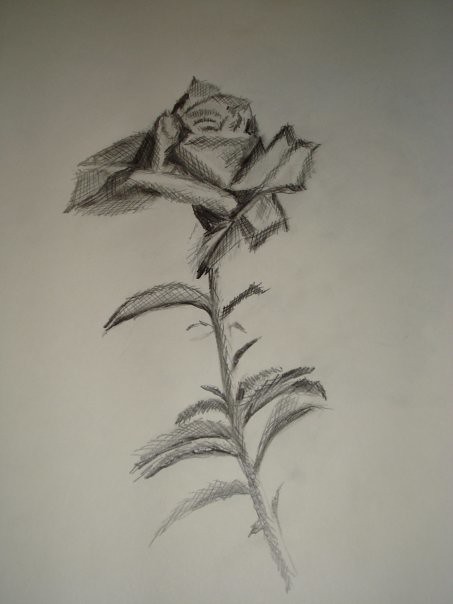This is a detailed photograph of a hand-drawn sketch, likely created using black and gray pencils, or even charcoal. The artwork, done on a plain white piece of paper oriented vertically, depicts a rose-like flower. The flower emerges from a single stem positioned at the center bottom of the paper. As the stem rises toward the center, it slightly curves, featuring several leaves on either side. The leaves vary in detail, with some appearing more pronounced, possibly even resembling thorns.

At the top, the flower's petals radiate outward, arranged in a somewhat angular manner, possibly creating an impression of a face within the petals. The sketch employs heavy shading, predominantly through crosshatching, supplemented by more deliberate strokes in certain areas. The background showcases a subtle gray gradient, darker at the top and lighter towards the bottom, potentially due to vignetting from the photograph. Some smudge marks and minor dirt around the edges suggest a natural, unedited capture of the drawing, likely taken with a camera phone. Despite the lack of color, the intricate details and shading emphasize the beauty and complexity of the sketched rose.